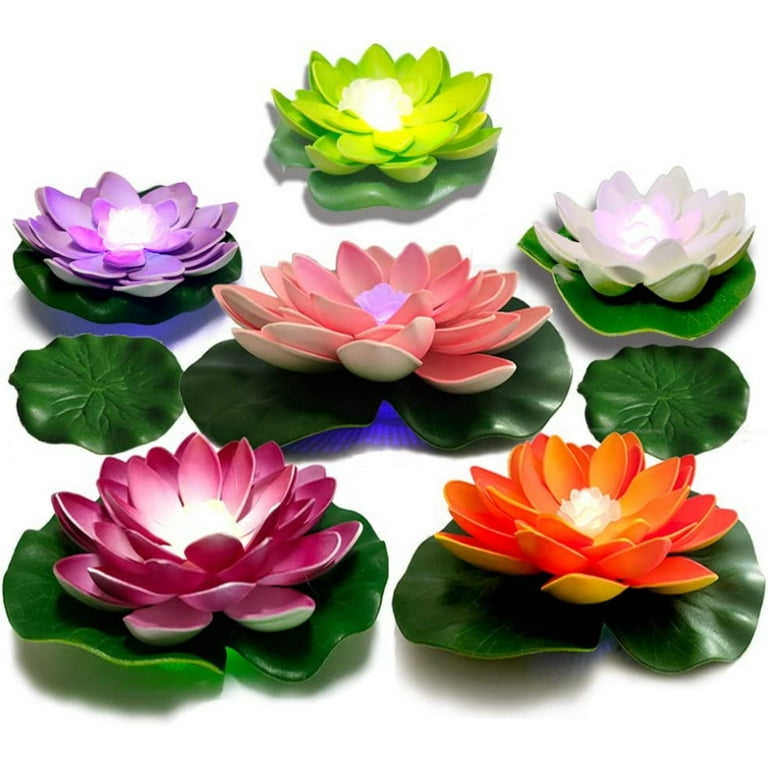The image features several artificial flowers laid on top of green lily pads. There are about six brightly colored flowers arranged among the lily pads, with two pads remaining empty. At the top center of the image, a vibrant green flower with a white center stands out. To its left, there's a purple flower with a white center, while to the right, you see a white flower with multiple petals, also bright at the center. Dominating the middle is a large peach or red flower with a purple core. The bottom left of the image features a dark pink flower with a bright center, and the bottom right displays an orange flower with several glowing petals. All the flowers, which resemble lotuses or succulents with sharp, pointy leaves, appear to be placed evenly across the lily pads, encircling the prominent central pink flower.